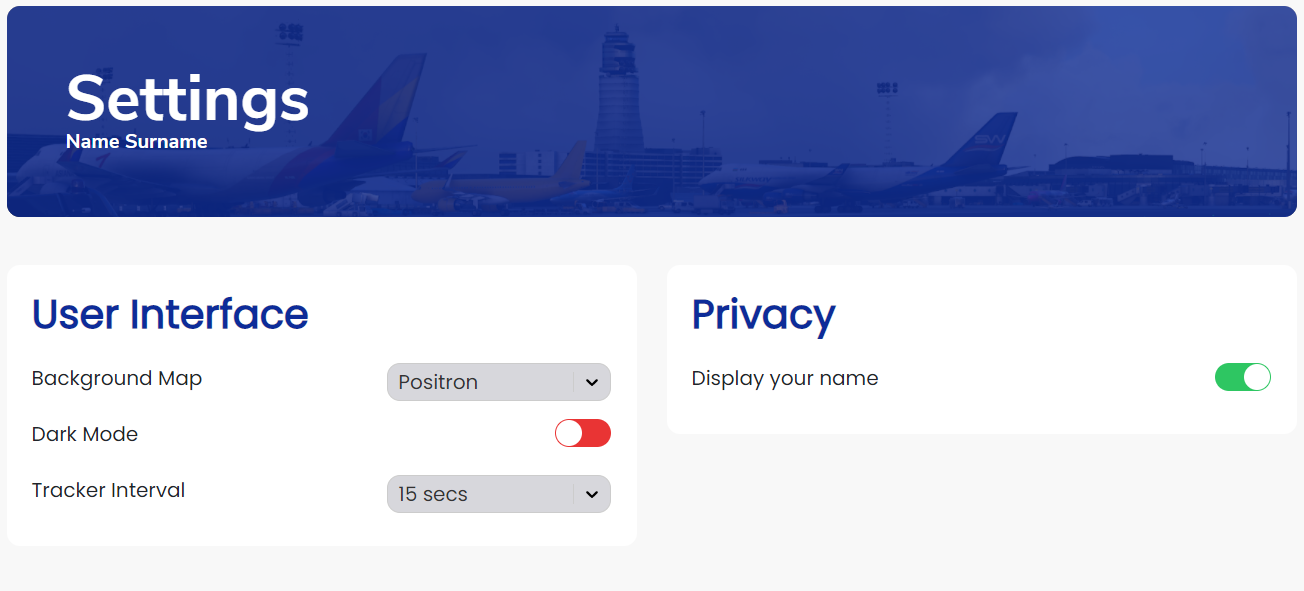Here's a revised and detailed caption:

"A screenshot of a settings menu from an airline's website. The interface features a prominently displayed blue navigation bar at the top, with a faint transparent image of a plane in the background. The title 'Settings' is prominently written in white lettering. On the lower left-hand side of the menu, there is a section labeled 'Name and Surname.'

Below this section, a blue bar is visible, under which the words 'User Interface' are written, also in blue. The background setting is identified as 'Positron,' and both 'Dark Mode' and 'Tracker Interval' settings are noted. 'Dark Mode' is turned off, while the tracker interval is set to 15 seconds. 

To access the 'Contacts' menu, there is a pull-down option available. To the right of this menu, a white bar displays the 'Privacy' section, highlighted in blue text. The setting to 'Display Your Name' is turned on.

Overall, this menu seems to pertain to the user and privacy settings for an airline booking website, offering users options to adjust their interface preferences and manage privacy settings."